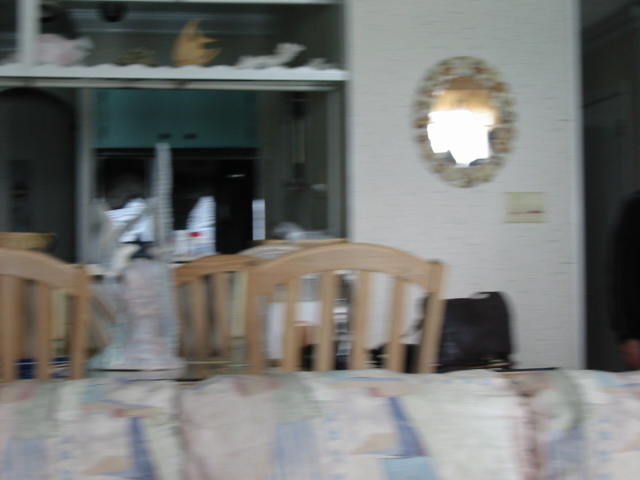This is a very blurry and dim photograph of the interior of a home, reminiscent of photos taken with old disposable Kodak cameras. The image captures a nostalgic, outdated living room. In the foreground, there is the top rim of what appears to be a multicolored couch in muted tones of tan, blue, and possibly maroon. Behind the couch is a glass-top dining table surrounded by three to four light blonde wooden high-back chairs. A white bust serves as a centerpiece on the table. The background reveals a white-painted wall adorned with a large, oval decorative mirror. Below the mirror, a cream-colored plastic light switch panel is visible. To the right, there is a small side table with a black purse. Further back, the kitchen can faintly be seen, marked by blue cabinets and shelves with decorative items. Additionally, there is a dark opening that leads to a hallway on the right side of the composition.